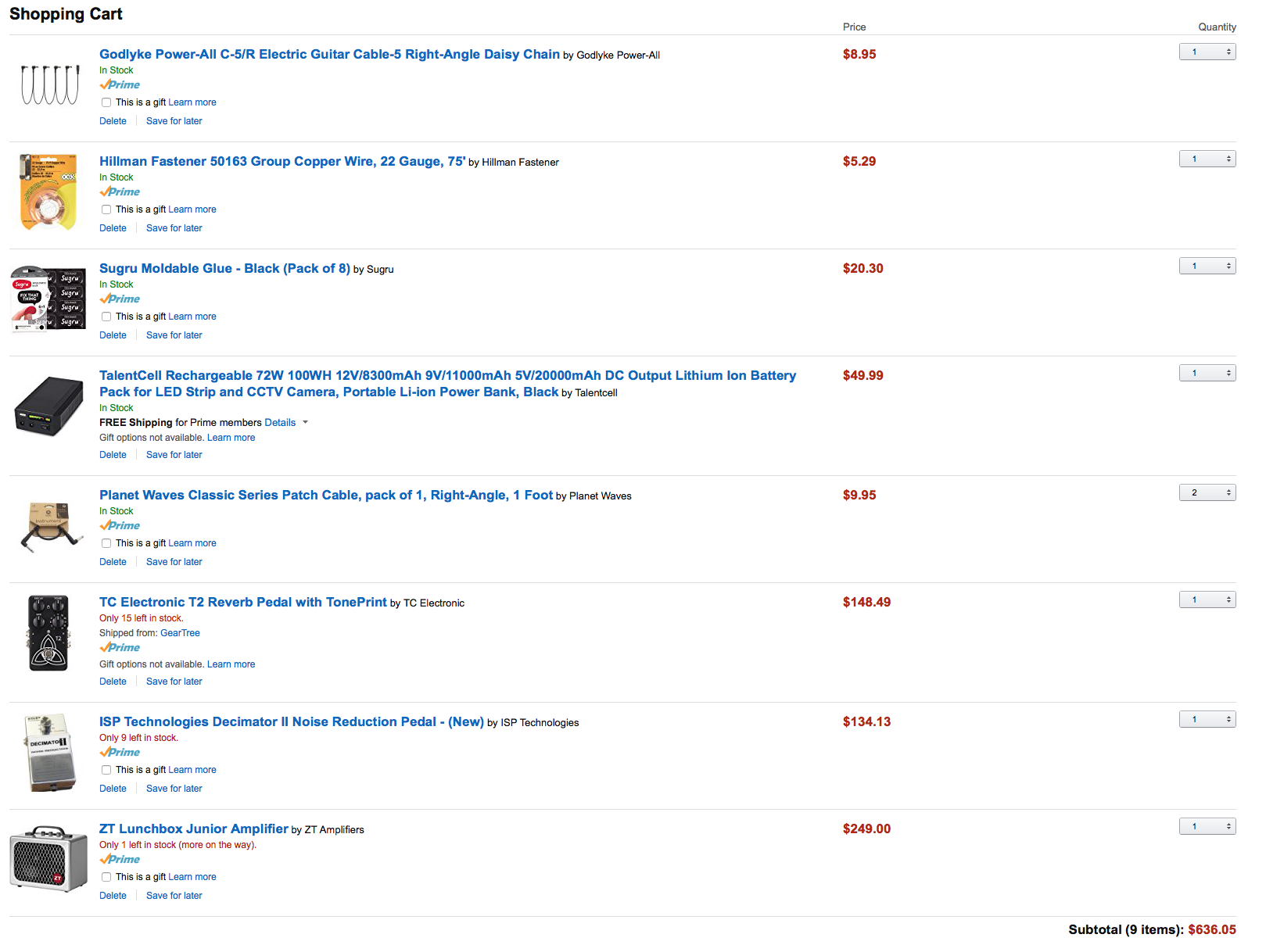This image is a screenshot of a shopping cart from what looks like a popular e-commerce platform, possibly Amazon, given the recognizable Prime logo. The image itself is wider than it is tall, approximately 20% wider.

At the top left corner, there's bold black text that reads "Shopping Cart," indicating the main section of the webpage. Adjacent to this, in the header area, are two more columns with much smaller, unbolded black font: "Price" positioned centrally, and "Quantity" aligning to the right.

The "Shopping Cart" column dominates about 60% of the page width and contains a list of items, each accompanied by an image to the left and a description in blue text. Below each item description, there is a Prime logo with a 'check' mark indicating that the item is eligible for rapid Prime shipping. Additionally, there are checkbox options labeled "This is a gift," followed by buttons for "Delete" or "Save for later."

There are eight items visible in the shopping cart list, including:
1. An electric guitar cable
2. A fastener
3. Some glue
4. A battery

The detailed layout ensures ease of navigation and clarity for someone managing their purchases, with emphasis on key features like item description, Prime eligibility, gift options, and item management actions.